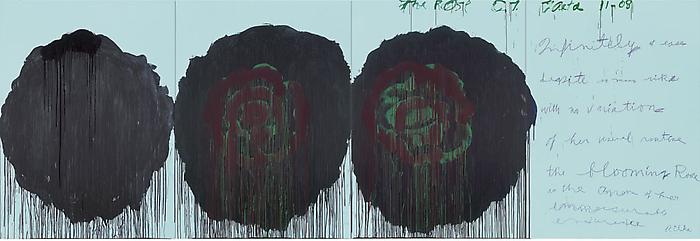This horizontally oriented painting features a background of light blue, with three prominent, circular or oval-shaped, dark grey to black blobs arranged from left to right. Each blob has delicate, dark fringes that drip downwards in vertical lines. The leftmost blob is completely dark, almost blending into black. The central blob faintly reveals a dark red rose at its core, while the rightmost blob clearly displays a rose with visible red and green hues, standing out more distinctly against the dark background. On the far right side of the image, in cursive text, are the words "11-8", "infinity" or "infinitely", "blooming", and other indecipherable words, perhaps reflecting an abstract, poetic theme.